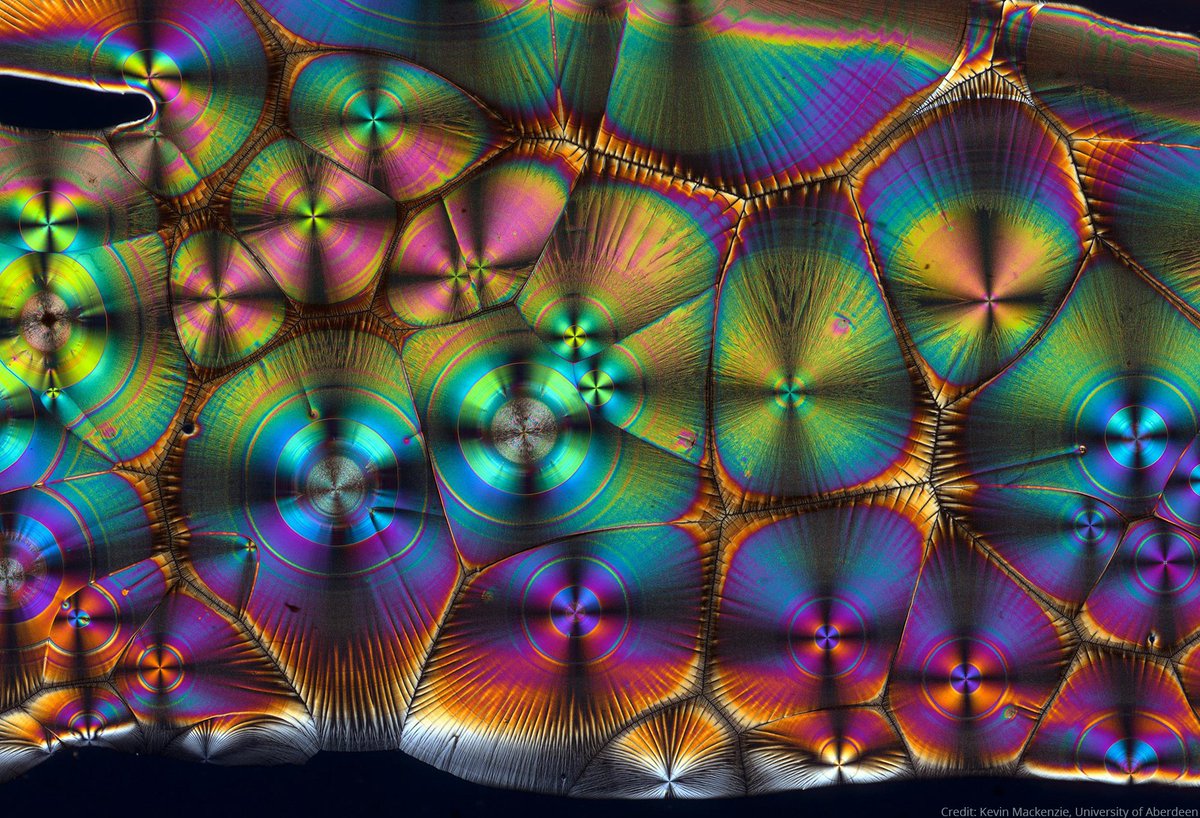The image showcases a mesmerizing, kaleidoscopic pattern against a stark black background. It features an array of vibrant colors, including purple, blue, green, yellow, orange, and pink, arranged in a fragmented and segmented manner reminiscent of looking through a kaleidoscope. The pattern consists of numerous circular and oval segments, some of which are distorted into shapes resembling rectangles or triangles. These segments are intricately joined together, evoking the texture of snake skin.

Each shape within the pattern displays a radial gradient, where colors transition from the edges to different hues towards the center. The image includes an assortment of distorted circles, ranging from very large to medium-sized, especially noticeable on the right and bottom sides, with smaller ones scattered throughout. The clustered shapes create a psychedelic effect, with prisms of green and yellow being particularly prominent. Rays of color extend across the top and bottom, adding to the dynamic, converging visual experience. The overall effect is a captivating spectacle of shapes and colors that seem to dance and morph as though viewed through the shifting lens of a kaleidoscope.